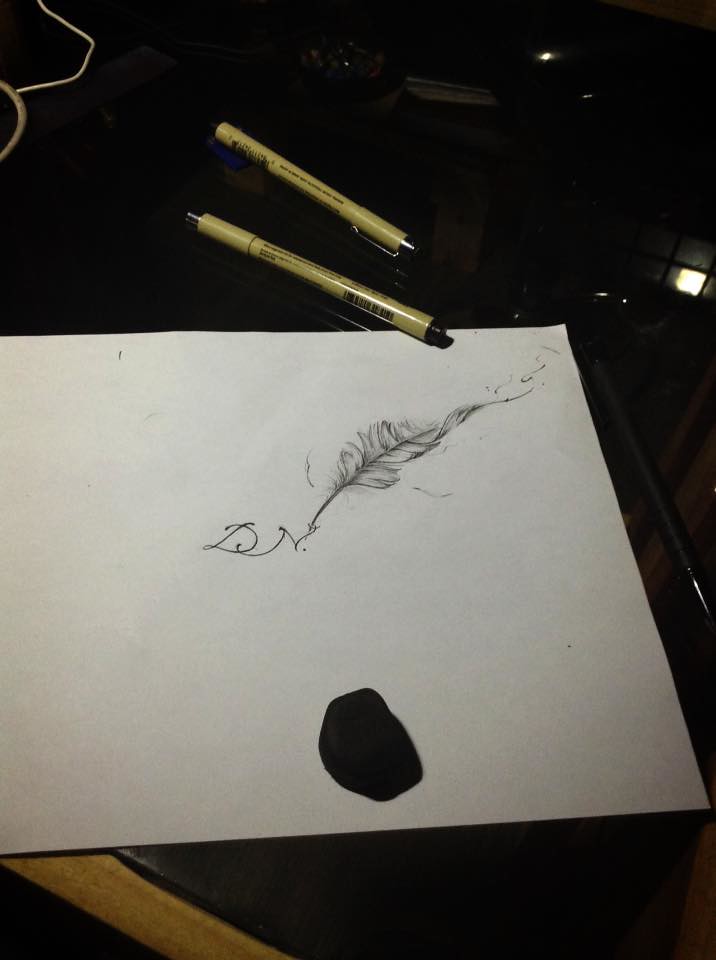The image depicts a white sheet of paper placed on a circular table with a black surface. Resting on this paper, there are several items meticulously arranged. In the upper section of the photograph, two pens are visible—one lies on the paper while the other is positioned farther up on the table. The central focus of the image is an intricately drawn quill pen. The quill's feather, rendered in fine detail with pencil strokes, contrasts against the simplistic, thin line representing the quill's shaft. This illustrated quill appears to be drawing or has drawn the initials "D N" on the paper. Additionally, a dark object is situated at the bottom middle of the image, partially intersecting with the paper, adding a contrasting element to the composition. The overall scene is rich in texture and detail, blending different materials and artistic mediums.